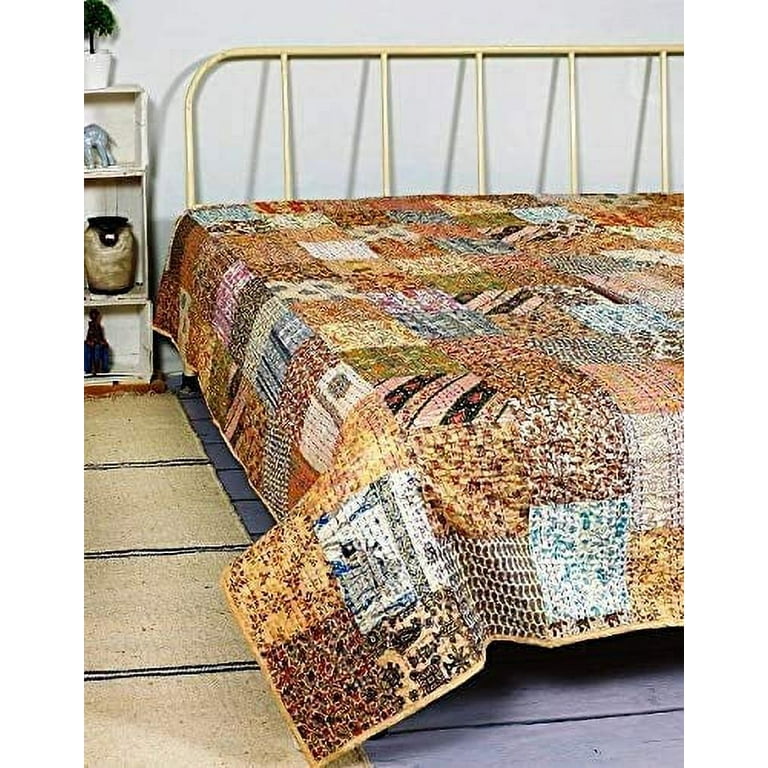This photograph showcases a vintage-style bedroom featuring a spacious bed adorned with a colorful, multi-patterned quilt. The bed's frame is composed of brass, adding to the old-fashioned charm of the room. Notably, there are no pillows on the bed. Adjacent to the bed on the left, there is a white bookshelf partially visible, hosting an artificial plant atop it and displaying a sculpture of an elephant and a vase on one of its shelves. The walls are painted white, further enhancing the room's classic aesthetic. The floor features two types of striped carpeting: one in tan and another in blue. The bed and the bookshelf extend beyond the frame of the image, creating a sense of continuity within the cozy, well-curated space.